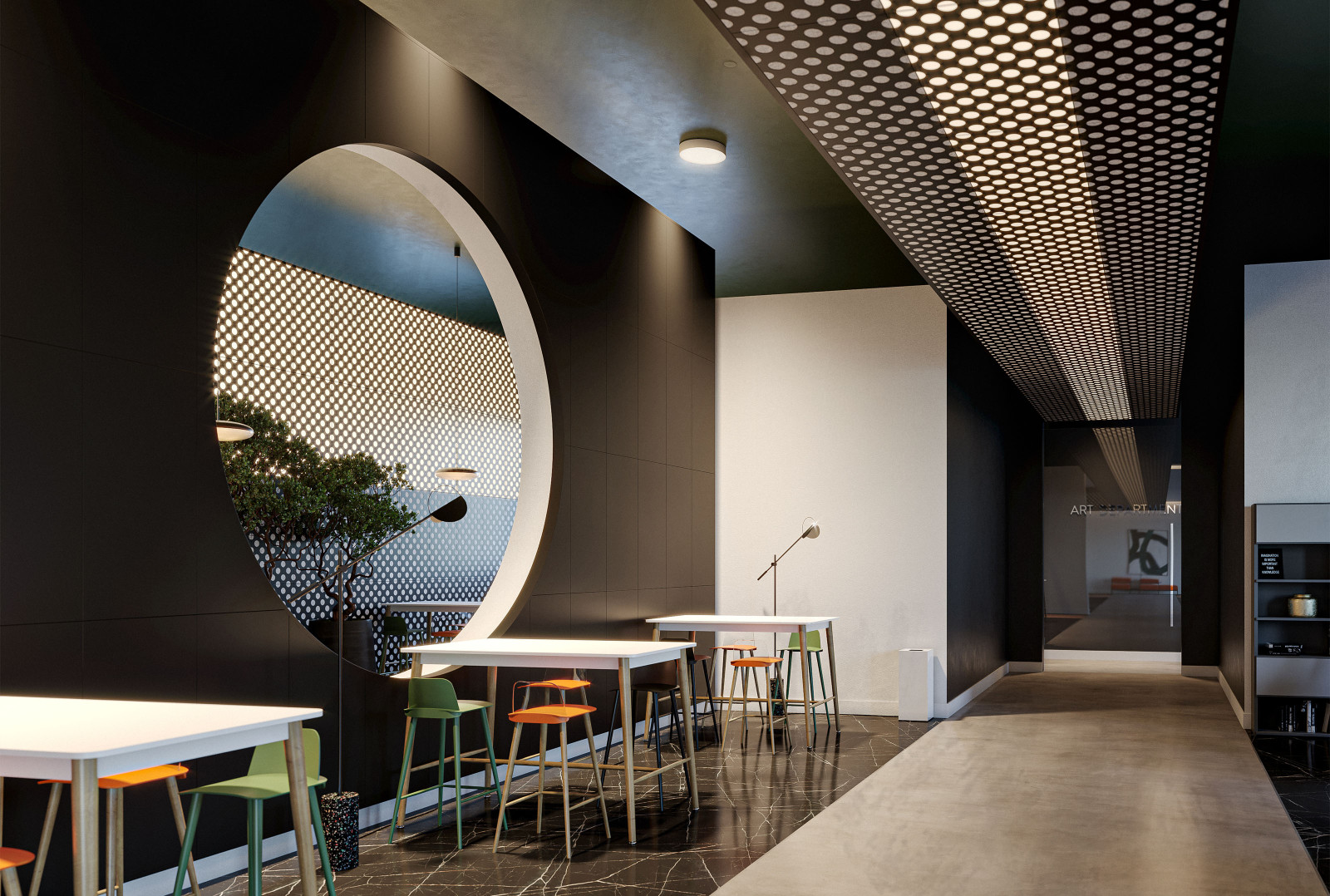This image portrays the interior of a clean, minimalistic cafe or college dining hall. The space is adorned with high top tables and stools in vibrant hues of orange and green, creating occasional pops of color against the otherwise monochromatic setting. A large window allows natural light to flood the room, complemented by a row of ceiling-mounted canister lights. The concrete floors and sleek furnishings lend a modern but somewhat uninviting atmosphere, lacking warmth and comfort. Despite the minimalist design, there's a hint of potential activity, as a microphone stand suggests a designated area for open mic performances or acoustic sets, reminiscent of nostalgic memories of intimate, albeit awkward, coffee shop gigs. The overall design prioritizes a clean and clear environment, ideal for studying or brief social interactions.